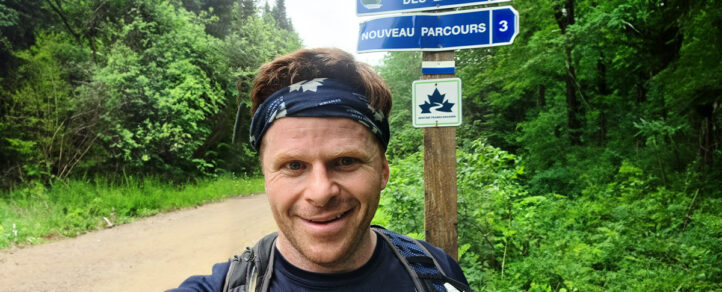A middle-aged, clean-shaven man is taking a selfie during his hiking adventure in a foreign country. He has a big smile on his face, revealing his excitement and pride, likely having just accomplished a significant milestone in his hiking journey. He is wearing a dark blue shirt, a backpack with blue straps, and a blue bandana adorned with small white leaves, which keeps his medium-length brown hair out of his face. The background features a lush forest with green trees lining either side of a brownish trail. Prominently behind him, there is a wooden post with two blue signs in white writing; the first sign reads "NOUVEAU PARCOURS," along with the number three, likely indicating a trail marker in French, and the second is a smaller white sign depicting three green leaves.